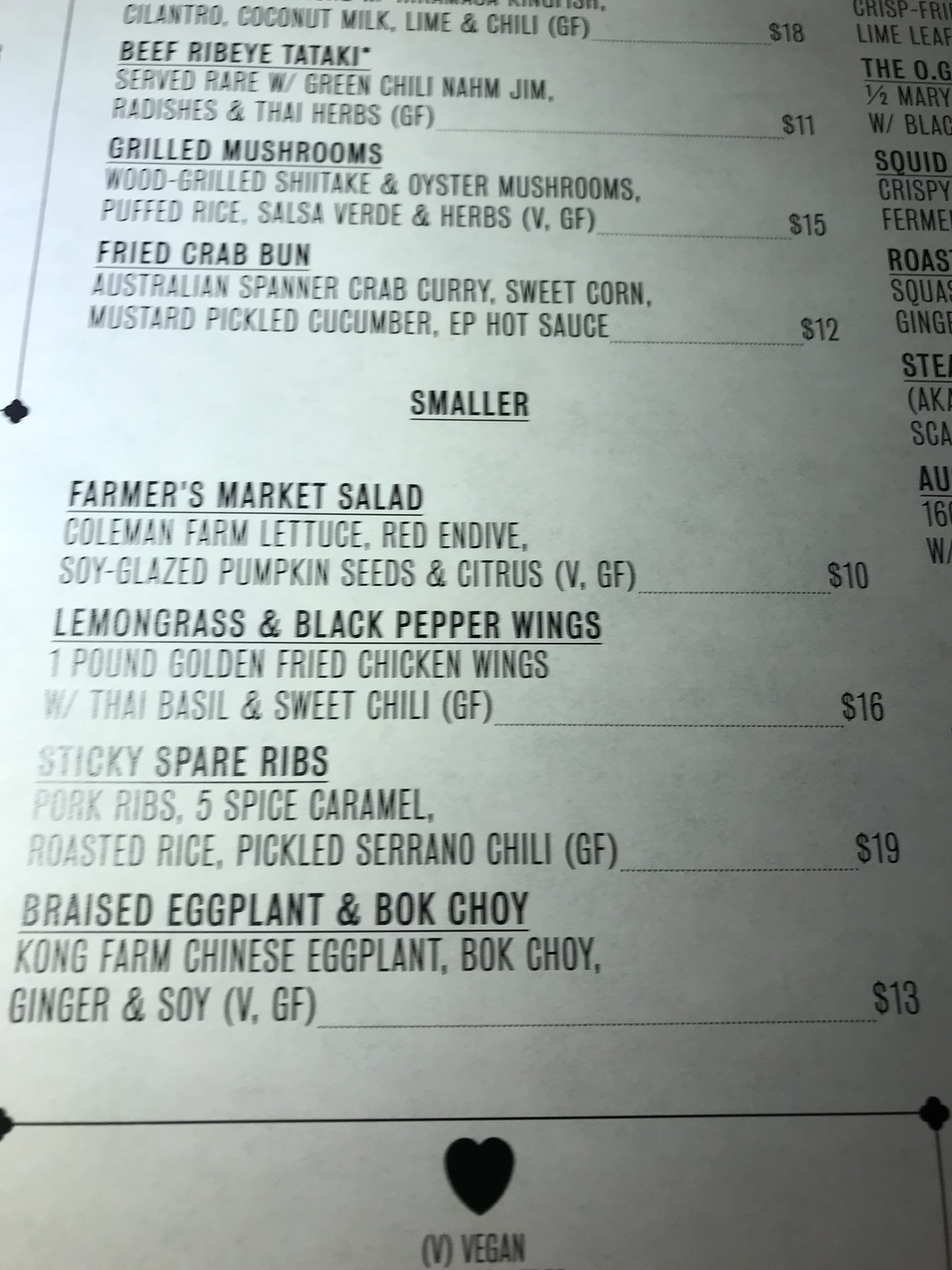This close-up photograph captures a detailed section of a restaurant menu. The menu is printed on white paper with black ink. The focus centers on one column, with a glimpse of another column just off the right edge. There is noticeable glare in the lower-left corner, likely from a flash. 

The upper portion of the visible column highlights items such as Beef Rib Eye Tataki, Grilled Mushrooms, and Fried Crab Bun. These item names are bolded and underlined, each accompanied by a brief description of the ingredients. Prices listed alongside these items are $18, $11, $15, and $12, respectively.

In the lower half of the image, a section is labeled "Smaller," both bolded and underlined, and centered. Items here include Farmer's Market Salad, Lemongrass and Black Pepper Wings, Sticky Spare Ribs, and Braised Eggplant and Bok Choy, with prices at $10, $16, $19, and $13 respectively. A horizontal line with diamonds at each end separates this section from the next. Below this line is a black heart symbol followed by the letter "V" in parentheses and the word "Vegan," indicating vegan options.